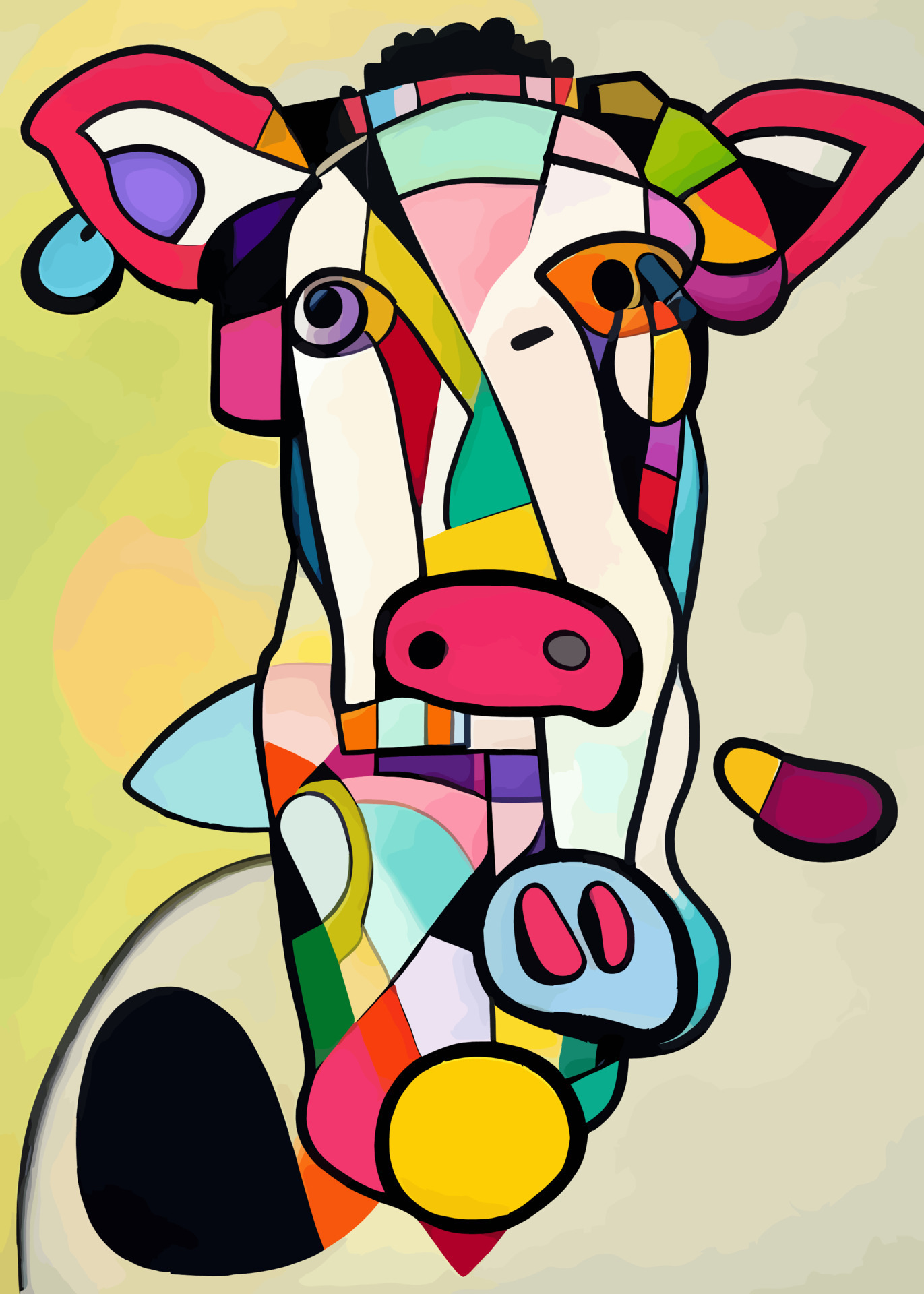This is an abstract painting reminiscent of Picasso's vibrant style, depicting a distorted, colorful cow against a beige or light green background. The cow's red ears, pink nose with black and gray nostrils, and mismatched eyes—one blue, the other orange with black—are prominently featured. The face tapers from the ears to the nose, suggesting the cow's head. The top of the head is painted purple. Notable details include a blue hoof with two red marks at the bottom, and a yellow globe with a black background beneath this hoof. In the bottom left corner, a swirl resembling a half-circle, white with a black mark, adds to the abstract quality. The body of the cow is distorted and fragmented into a mosaic of various colors including pink, blue, white, green, purple, orange, light blue, and beige, creating a stained-glass effect. The painting exudes a feverish energy through its vivid palette and distorted shapes, emphasizing the abstract nature of the composition.